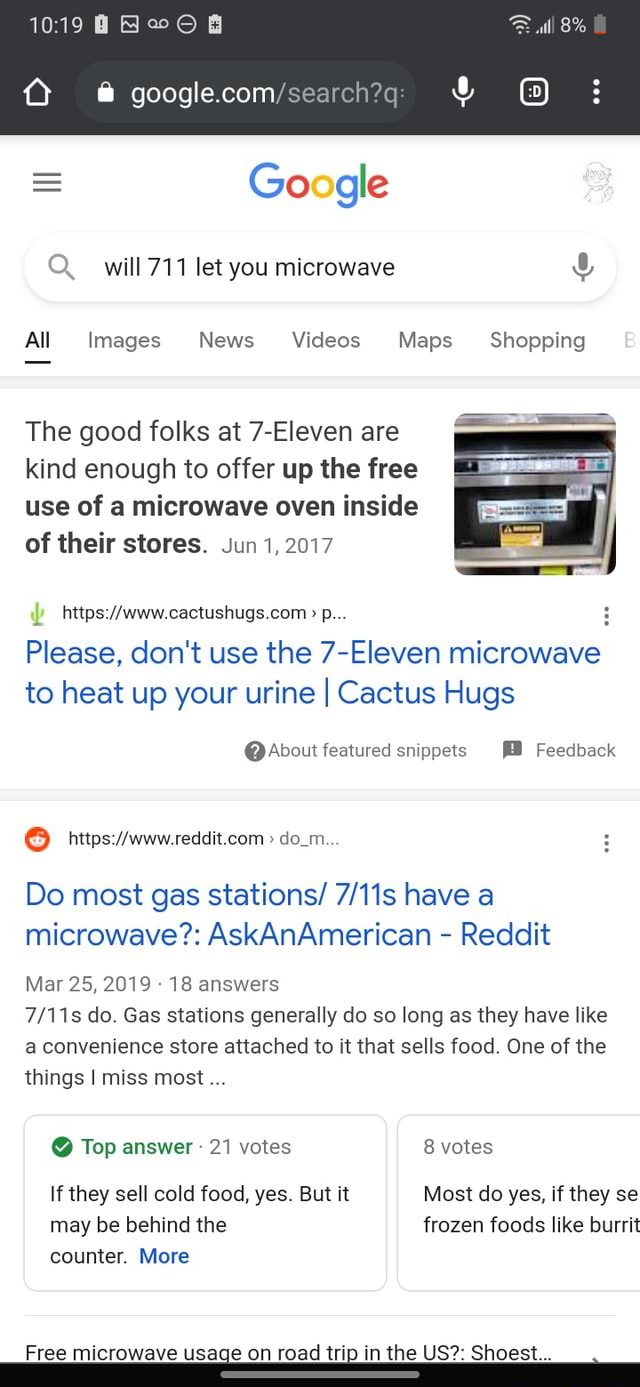The screenshot appears to be from an Android phone displaying a Google search results page. The time on the top left indicates 10:19, and the battery meter, located on the right, shows an exclamation point with the battery level at 8%. The Wi-Fi signal is at full strength, while the cellular signal is 4 out of 5 bars.

Just below the status bar is the Google search URL bar, displaying "google.com/search?q=" with a house logo to the left and a microphone icon on the right. Further to the right, there is a square icon for viewing open tabs and a vertical three-dot menu icon for settings.

The main body of the screenshot, set against a predominantly white background, features the Google logo at the top center. To the left of the logo is a settings icon with three horizontal black lines. Next to the logo on the right is a grayed-out illustration of a waving boy.

Below this is the Google search input field with the query: "Will 7-Eleven let you microwave?" The first search result reads: "The good folks at 7-Eleven are kind enough to offer up the free use of a microwave oven inside of their stores." This result is dated June 1, 2017.